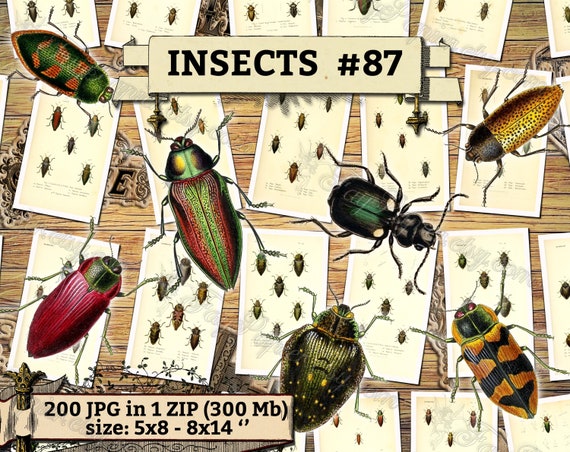This image is a detailed digital illustration titled "Insects Number 87" and features a collection of insects represented as playing cards. The illustration has a rustic, natural aesthetic with a background designed to resemble a wooden surface. At the top, a tan banner displays the title "Insects Number 87" in black lettering.

The main focus of the image is a spread of playing cards, each meticulously illustrated with various insects. The cards are numbered similarly to traditional playing cards, ranging from 1 to kings. These cards have a cream-colored backdrop and depict an assortment of beetles, each uniquely colored and patterned. Among the beetles, one is vibrant red, another has gold and brown spots, and another has a leafy-shaped body. There are also beetles with gold and black stripes, and deep green and black hues.

Overlaying these cards, larger and more detailed images of the insects are drawn, creating a layered effect. Each insect is carefully rendered, showcasing the artist's attention to detail and coloration.

At the bottom right corner of the image, another tan banner provides additional information: "200 JPG in one zip (300 MB). Size 5 x 8 - 8 x 14 inches." This text indicates the availability of the digital graphic as a collection of JPEG files, packaged in a ZIP file with a total size of 300 MB.

Overall, the illustration combines the structured format of playing cards with the organic beauty of insect life, all set against a backdrop that enhances its natural theme.